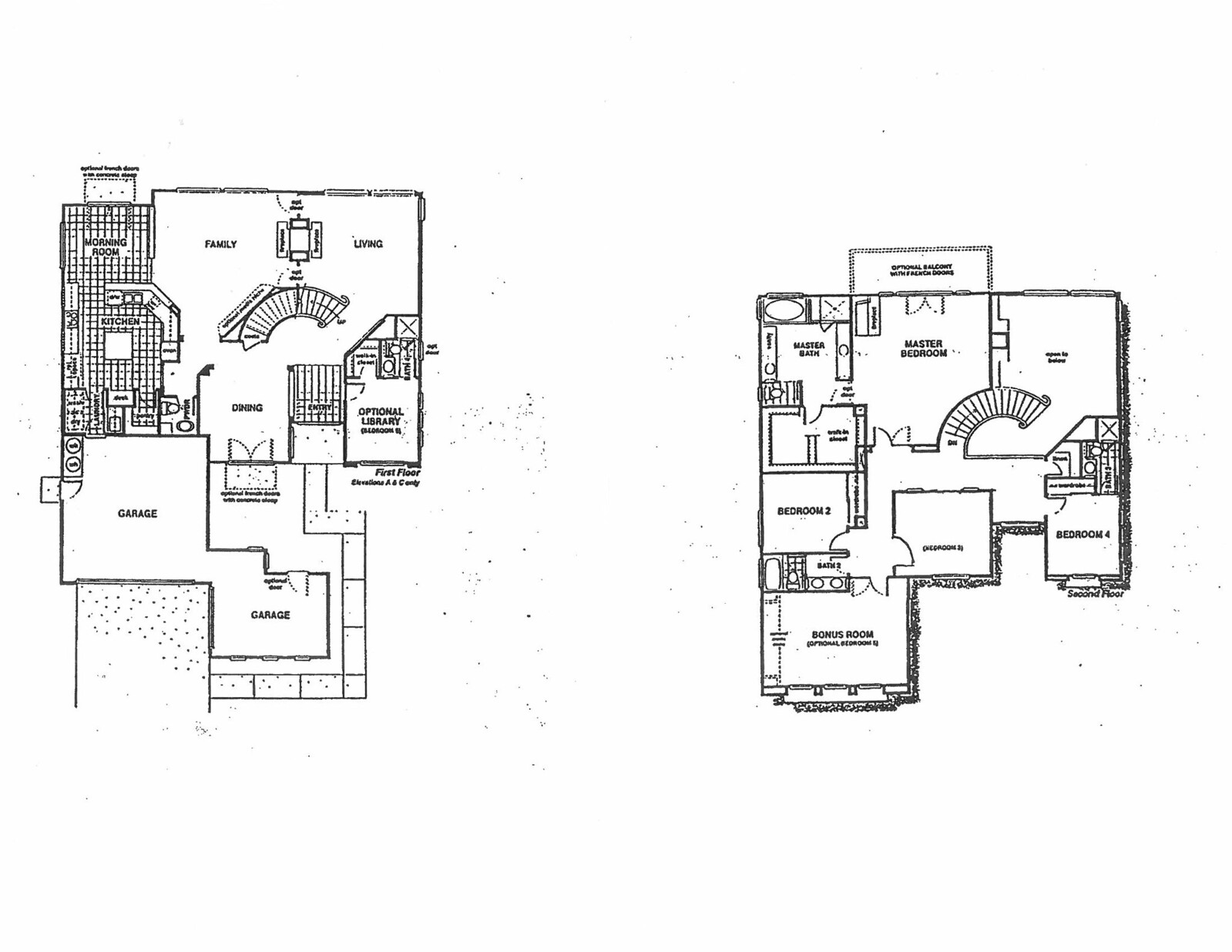The image showcases detailed floor plans, divided into two sections for the first and second floors. The first floor features a spacious family/living room with a detailed drawing suggesting a possible connection between the two areas. Adjacent to the family room is a circular staircase leading to the upper level. Across the hallway from the family living area, there is a dining room and an intricately depicted kitchen, which includes a morning room. The kitchen layout is notably detailed, with squares representing various elements on the floor. 

Connected to the kitchen, there is a garage which leads to another garage through a hallway. There is an additional room near these garages, though the small print makes it difficult to identify its purpose. 

On the upper floor, the circular staircase ascends into a hallway with a master bathroom, including specific features like a jacuzzi and a shower. This level also comprises four additional bedrooms, and details of a bonus room situated between the second and third bedrooms. This bonus room appears to be flexible for future use or expansion.